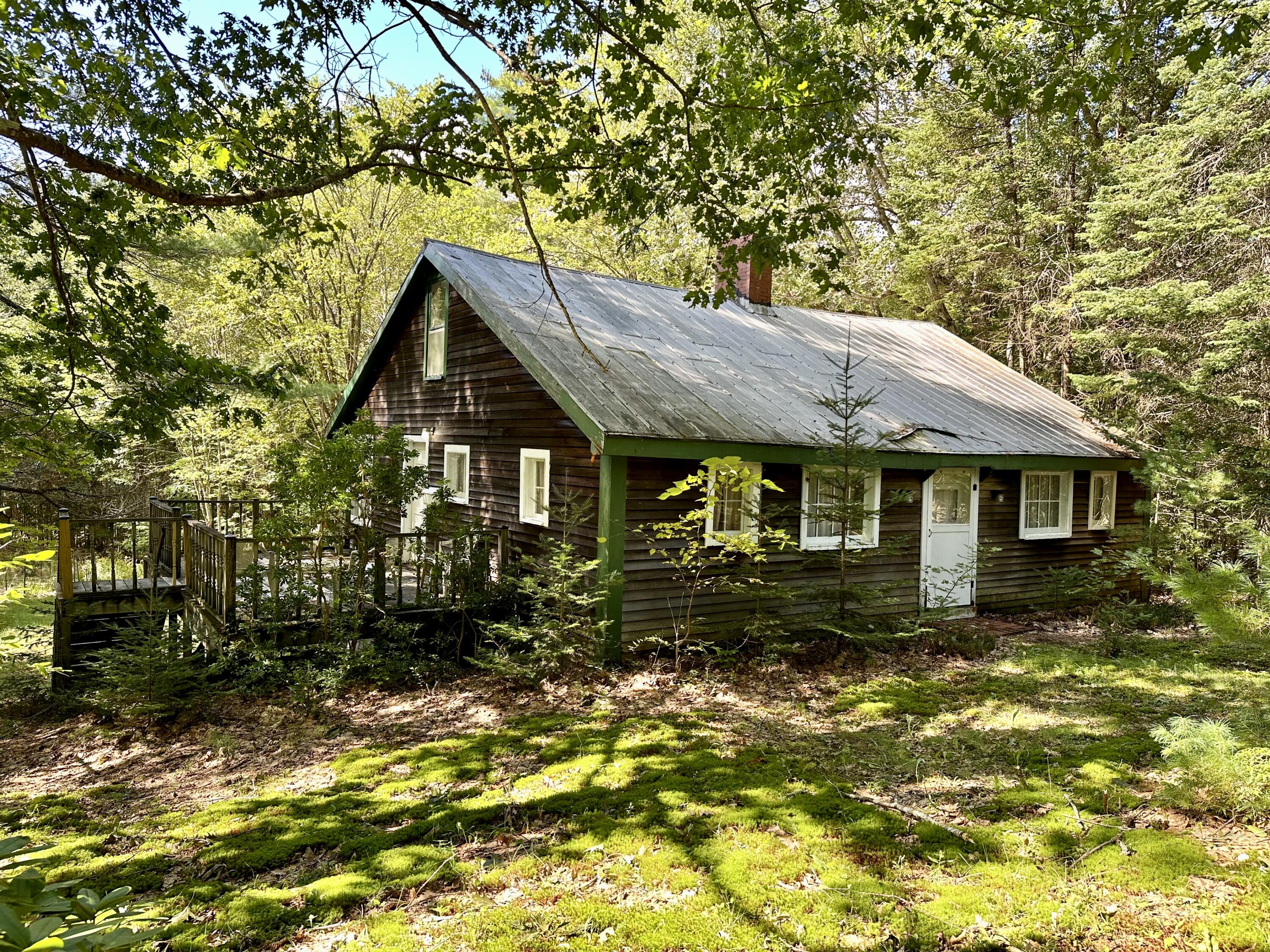The image showcases an older, cottage-like house situated in a heavily forested area, enveloped by various trees, including green pines and deciduous types. The house features dark brown siding, a silver roof with a touch of moss, and green fascia and trim around its edges, accentuated by white trim around the multiple windows and solid white doors. Central to the roof is a brown chimney. The front deck, matching the brown hue of the house, is partially engulfed by surrounding vegetation, with trees nearly encroaching onto it from the left side. Mossy grass carpet covers the ground, contributing to the overall untamed and rustic appearance, emphasizing that the property is not well-maintained. The scene, captured during the daytime, gives a sense of seclusion and wilderness.